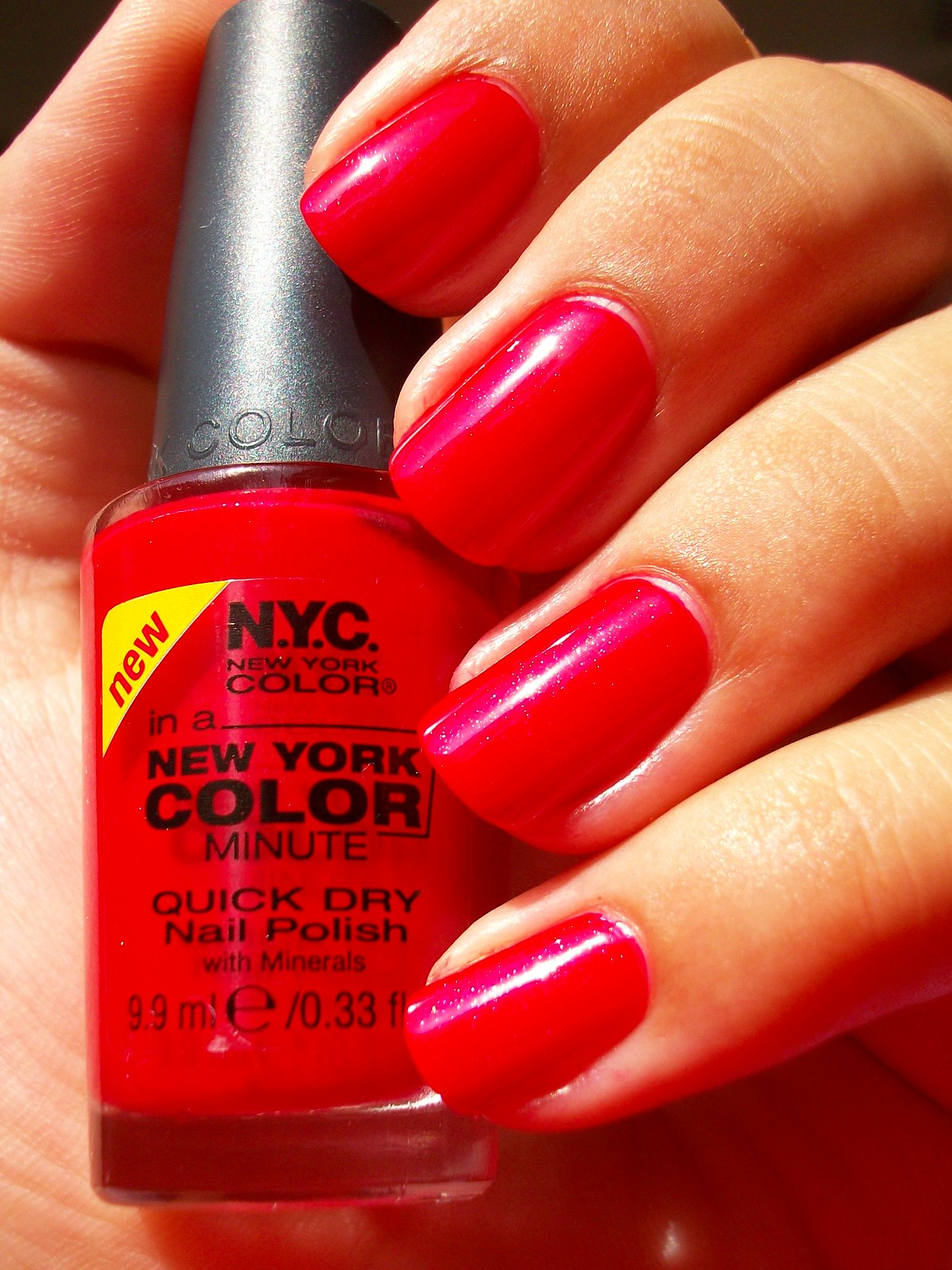A close-up image showcases the manicured hand of a Caucasian female, elegantly holding a bottle of nail polish. The nails are painted in a vibrant, deep red shade, emphasizing the polish being advertised. The bottle, which she holds with her thumb and has each finger wrapped around it, features a black cap with bold white text that reads "color." The nail polish bottle has a bright red base and is detailed with the text "NEW" prominently displayed in a yellow half-triangle on the upper left corner. Below, it reads "NYC New York Color" and "In a New York Color Minute Quick Dry Nail Polish with Minerals, 9.9 ml / 0.33 fl oz." The photograph, radiating a festive vibe, particularly fitting for occasions like Valentine's Day or Christmas, effectively highlights the product's sparkling red hue and quick-drying feature, making it an excellent advertisement.